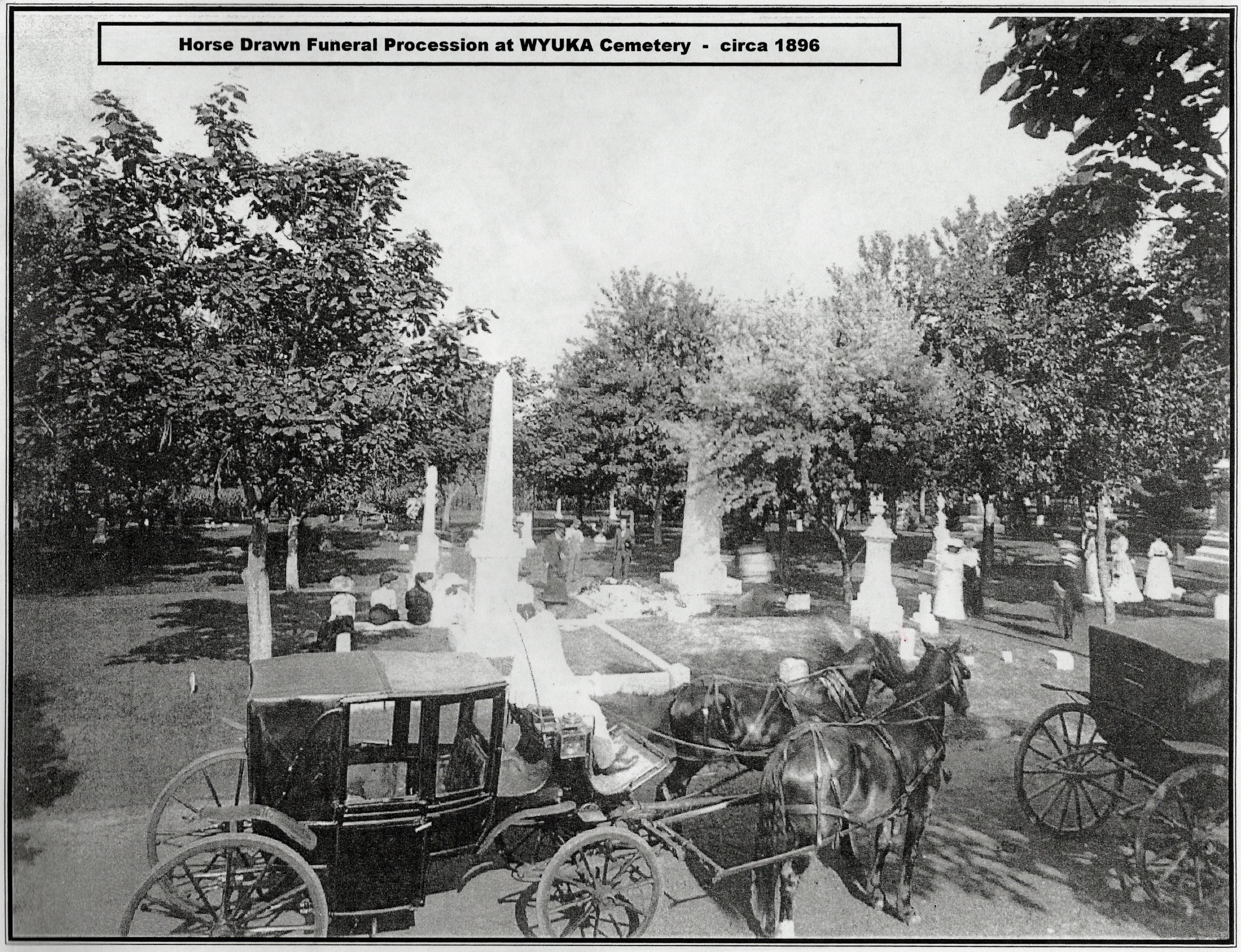This detailed black-and-white photograph, taken outdoors in 1896, depicts a somber horse-drawn funeral procession at WYUKA Cemetery. In the foreground, an old black carriage with large wooden wheels is prominently visible, led by two dark-colored horses harnessed to it. A person dressed in white is seated at the front, appearing to guide the horses. To the right of this carriage is another, though the horses pulling it are off-screen. The backdrop reveals a cemetery setting, characterized by a dense array of trees, stone monuments, and gravestones of varying sizes, creating an antiquated and poignant atmosphere. Scattered throughout the scene are blurred figures, some standing and some seated, likely mourning or attending the procession. Overhead, a black-outlined text box in the sky reads, "Horse-Drawn Funeral Procession at WYUKA Cemetery, circa 1896," grounding the historical context of the image. The photograph's timeless quality is underscored by its monochromatic palette, lending a nostalgic and respectful tone to the scene.